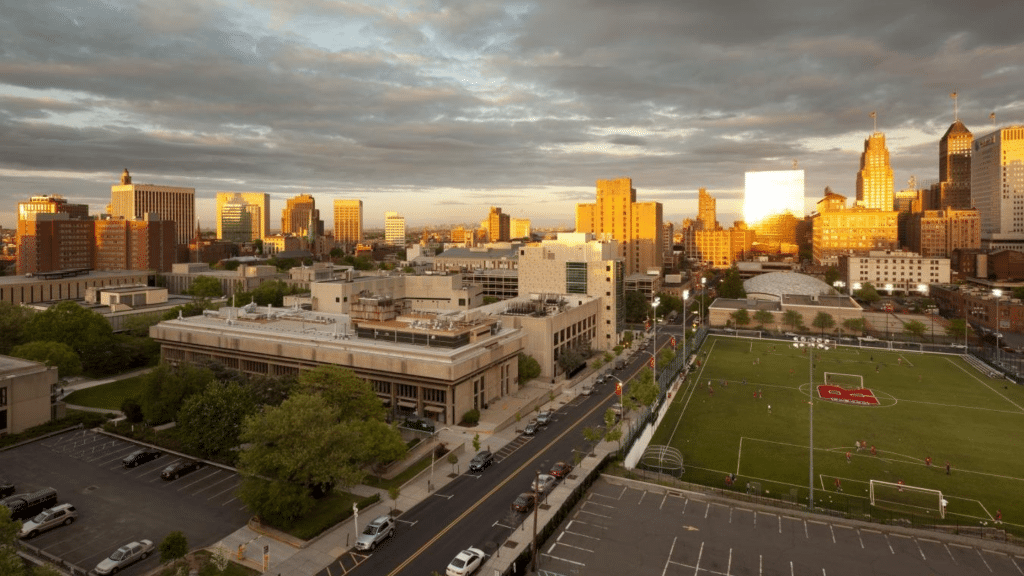A panoramic view captures a serene and relaxed cityscape at what appears to be evening or sunset. The skyline in the far background is adorned with an array of skyscrapers and large downtown buildings, with clouds vividly stretching across the sky. The middle ground features a prominent soccer field with lush green grass, prominently marked with a big red "R" in the center and bordered by white lines, all illuminated by stadium lights. Adjacent to the field, a few players are potentially practicing. 

In the immediate foreground, a light tan office building stands out, accompanied by a sparsely occupied parking lot. Across the street, lined with parked cars in various colors, stands what looks like a manufacturing plant or industrial facility, further adding to the city’s diverse landscape. Scattered trees are visible throughout, adding a touch of nature to the scene. Overall, the city exudes a peaceful ambiance, with ample open space and minimal traffic on the streets.